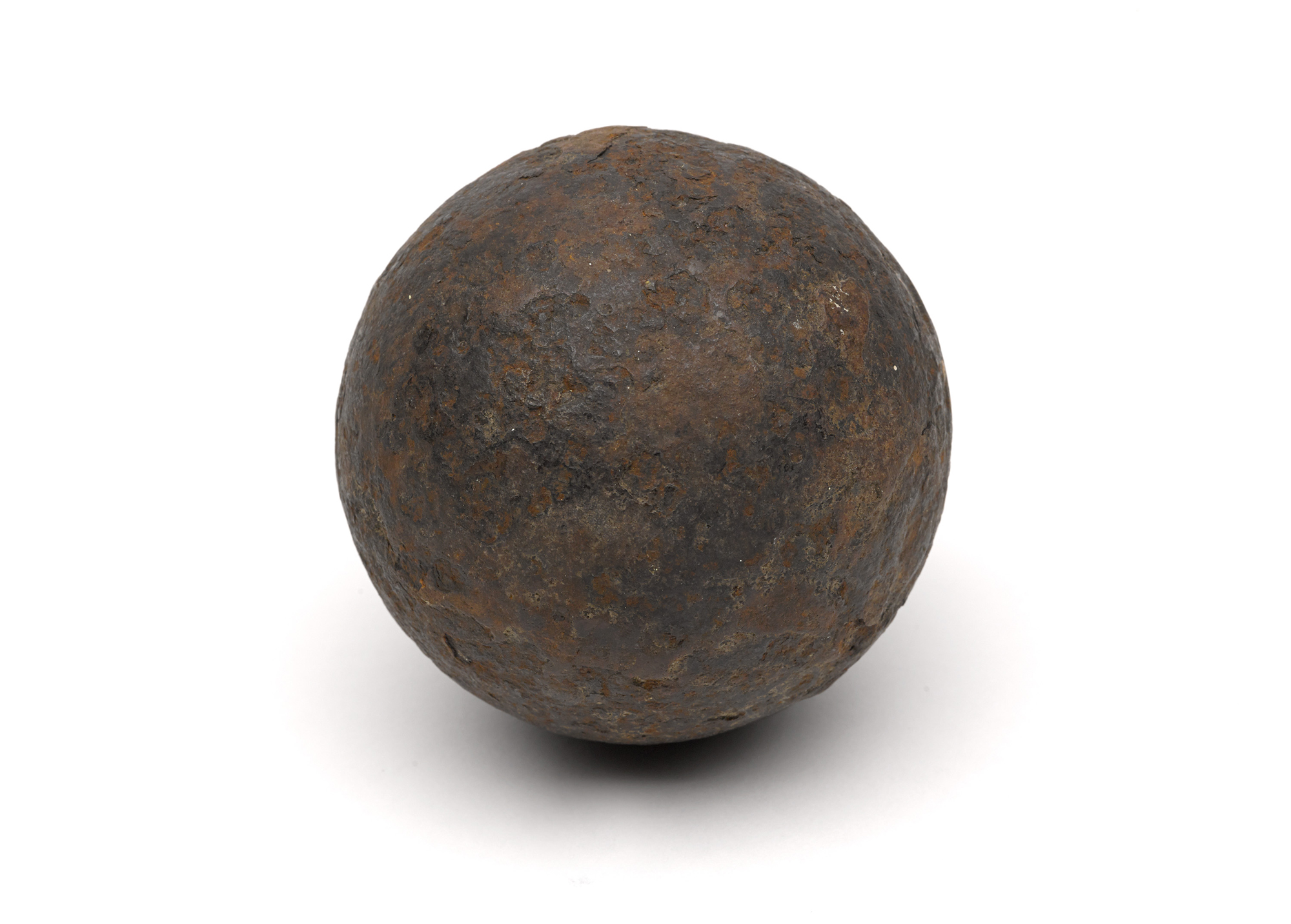The image is a detailed, close-up photograph of an old, rusted cannonball made of iron. Centered in a stark white background, the ball casts a subtle shadow directly beneath it. The cannonball exhibits a deep, uneven rust patina, characterized by a range of brown and black hues and a rough, flaking surface texture. The sphere, likely weighing around nine to ten pounds, shows no visible text or marks, just the natural patterns of oxidized metal. It evokes a historical artifact, reminiscent of a time when such objects were fired from cannons, now aged and corroded from years of exposure.